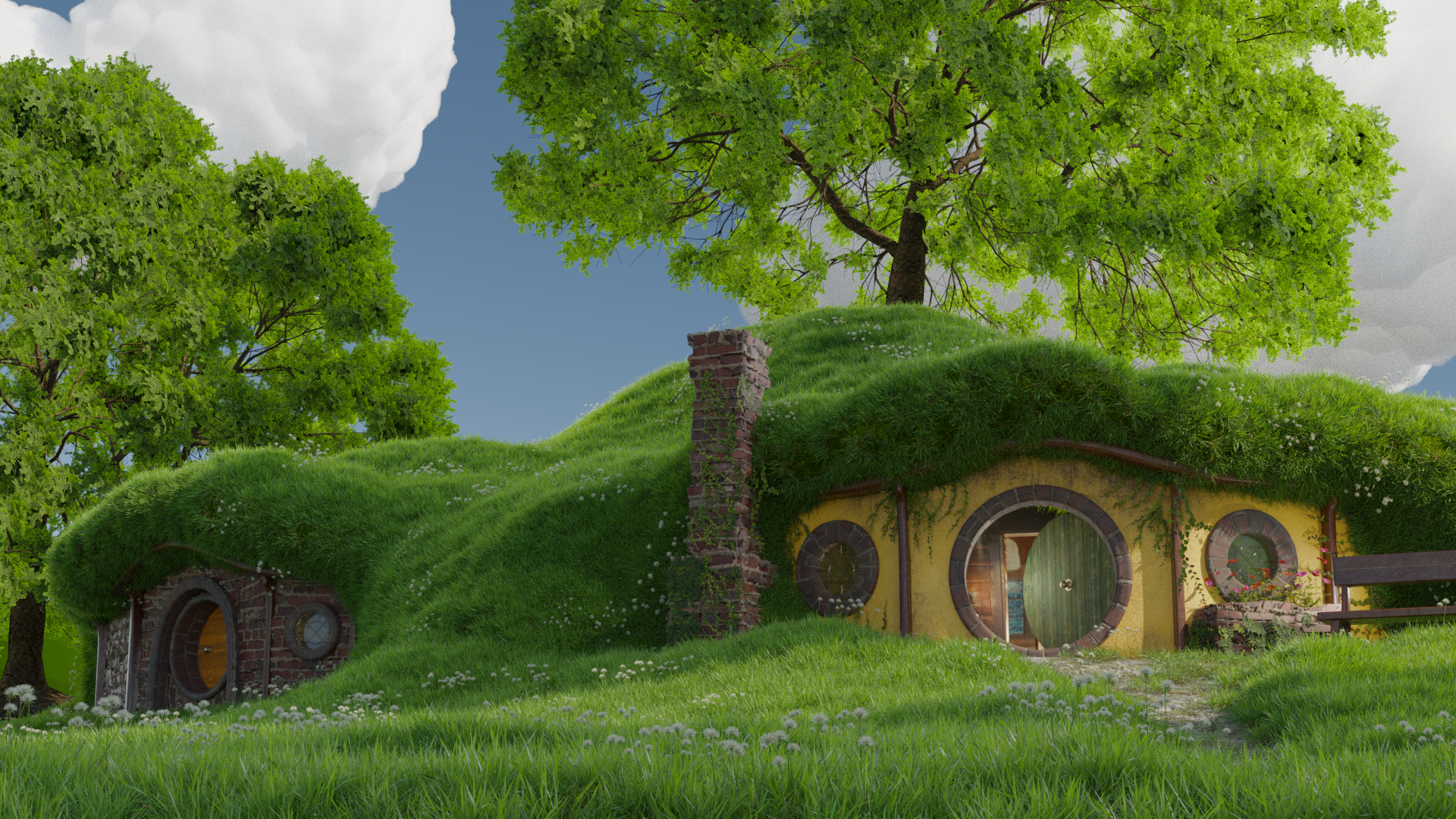Nestled within a small, grassy mound reminiscent of a scene from "The Lord of the Rings," this charming underground house boasts a whimsical design. A circular wooden door with a gold doorknob marks the entrance, surrounded by an exterior wall painted a cheerful yellow. The wall features a large circular window flanked by two smaller windows, all framed with brick. The roof is an earthy blend of dirt and moss, dotted with delicate blue flowers, seamlessly blending the house into its natural surroundings. A brick chimney peeks out from the roof, and two tall trees stand majestically behind the home, their branches extending protectively overhead. The sky above is a clear blue, with large, fluffy white clouds adding to the picturesque setting. To the right of the entrance, half of a quaint bench seat can be seen, inviting visitors to sit and take in the serene, storybook-like scenery.